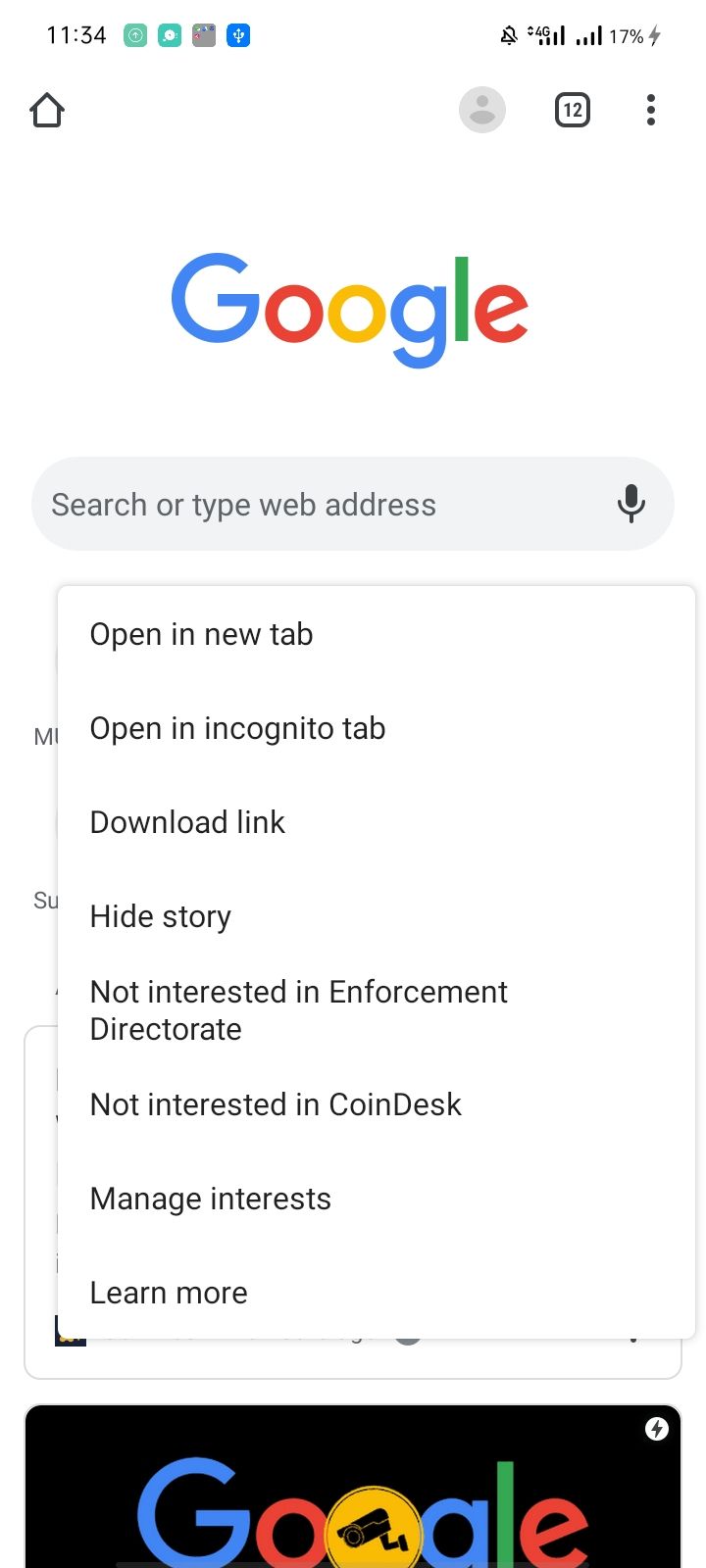The image depicts a smartphone screen displaying the Google homepage, characterized by its distinctive interface elements. At the top of the screen, the time reads 11:34, and the battery indicates a remaining charge of 17%. The Google search bar is prominently featured in the center, accompanied by a microphone icon for voice search functionality. The search bar itself is currently empty. Additionally, a pop-up menu is visible, presenting options such as "Open in new tab," "Open in incognito tab," "Download link," "Hide story," "Not interested in Enforcement Directorate," "Not interested in CoinDesk," "Manage interests," and "Learn more." Below this, the Google logo is displayed against a black background, maintaining its classic color scheme with an intriguing twist—a security camera is whimsically incorporated into the second 'O.' This may suggest a focus on security or surveillance themes. The home button is also visible, indicating the user can navigate back to their main screen.